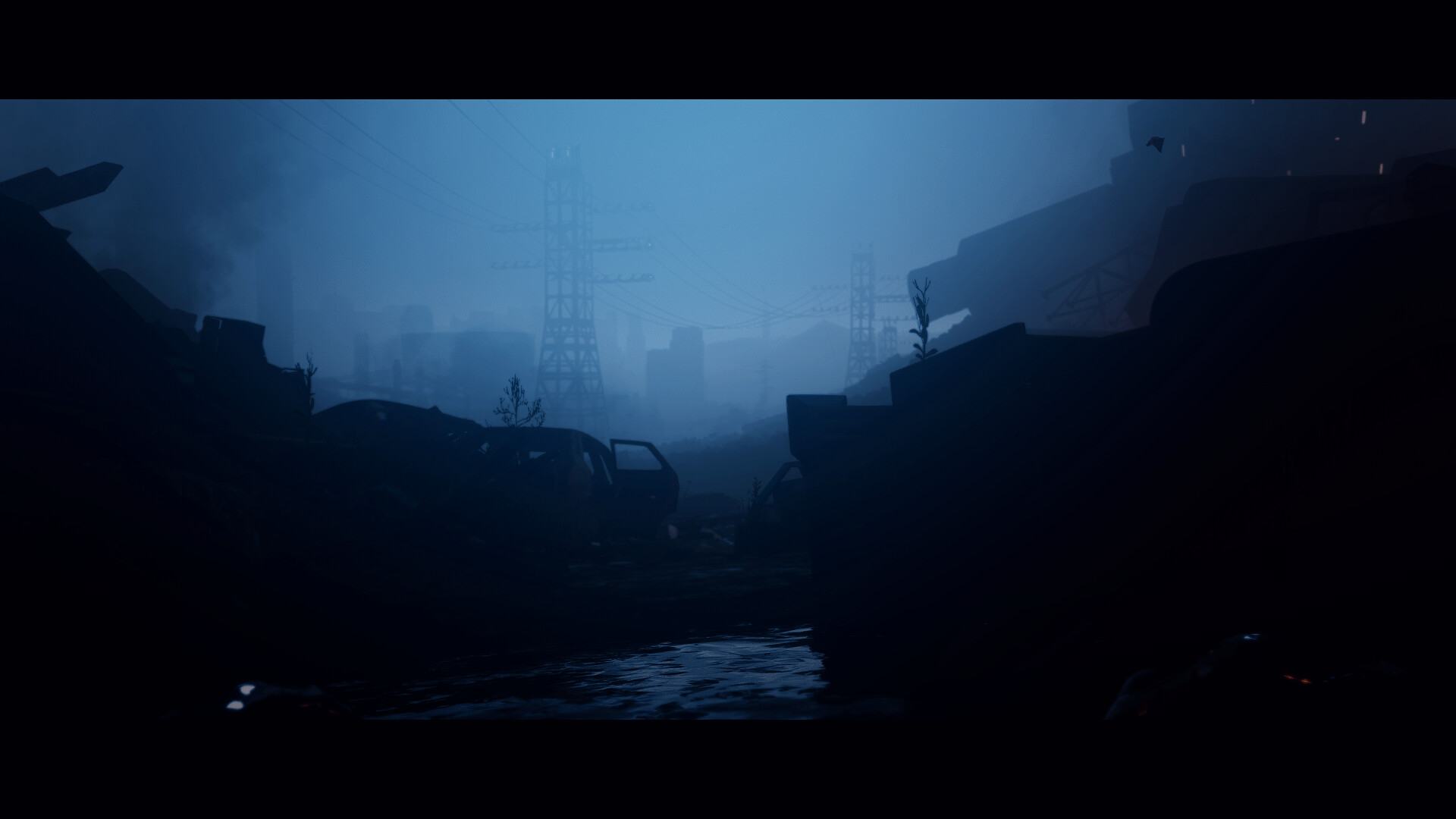The image depicts a dark, post-apocalyptic scene set in what appears to be a foggy or devastated junkyard. Dominating the background are the silhouettes of distant buildings and large metal electrical towers carrying power lines, giving a vague impression of a city masked by fog. The entire scene is rendered in monochrome shades of gray, amplifying its ominous, dystopian atmosphere. In the foreground, there's the outline of a car with its door open, possibly amongst other discarded cars and debris, indicating a junkyard setting. A patch of what could be snow or reflected light lies at the center, drawing the eye amidst the otherwise dark terrain. Tiny specks of white on the left suggest reflective material, while sparse vegetation is visible near the central vehicle. The right top corner also hints at more shaded buildings, adding to the overall sense of desolation.